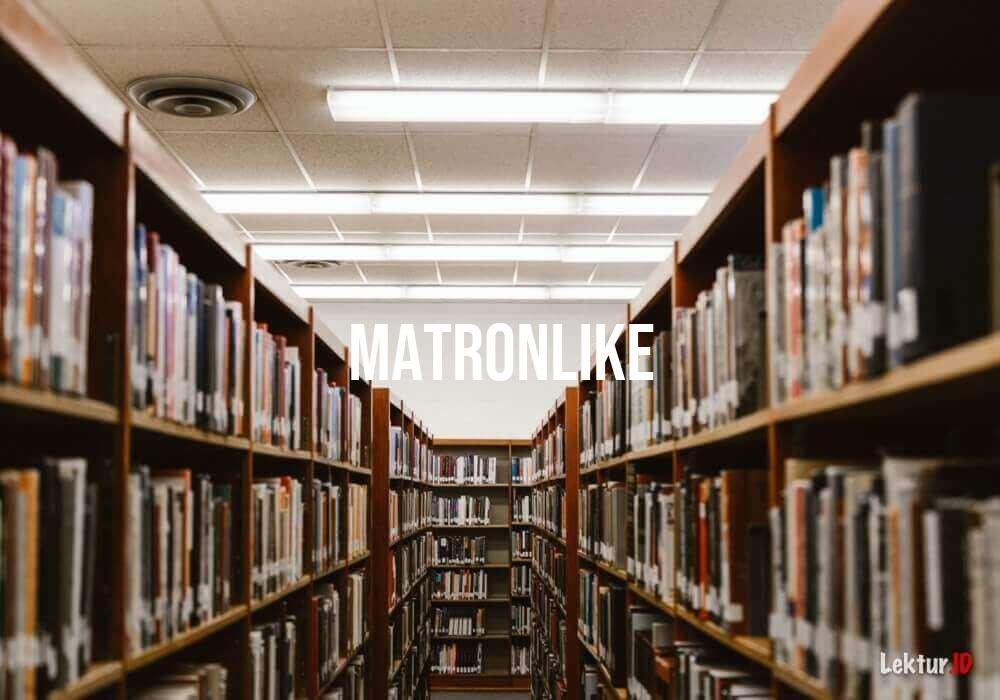The indoor, photographic image captures the view from a high vantage point, likely from a ladder, within a library. The scene features two parallel rows of brown wooden bookshelves, each filled with books. At the end of these rows is a wall of additional bookshelves, creating a vanishing point. The shelves and books are variously colored, predominantly brown, but also display blue, orange, and green hues. The ceiling is a dropped panel ceiling equipped with four horizontal fluorescent strip lights and a circular vent fan. In the center of the image, white text overlays with the words "Matron Mike." In the bottom right corner, the text "Lecter" (L-E-K-T-E-R) appears in white, and next to it, the red initials "J-O" are visible. The image is rich in detail, capturing the orderly linearity of the library’s architecture and its well-stocked shelves.